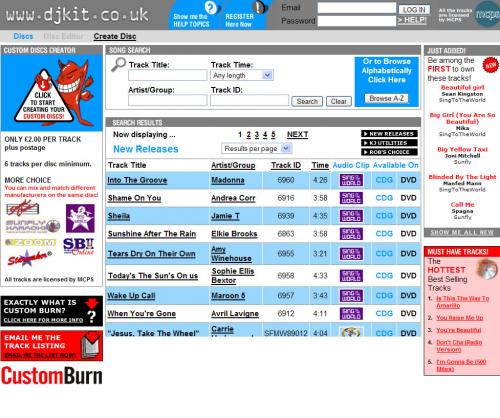This image is from the website www.djkit.co.uk. At the top, a grey bar serves as the banner, containing fields for email and password login. Beneath the banner, there is a section dedicated to creating and managing disks. On the left, a box features a devilish character holding a triangle with the text "Click to start creating your custom disks" inside it. 

To the right, in the center of the image, there is a section labeled "Song Search" where users can search for tracks by title, artist group, track ID, and time. Below this search box, a list of tracks is displayed with columns for track title, artist group, track ID, and duration. The first track on the list is "Into the Groove" by Madonna, with a duration of 4 minutes and 26 seconds.